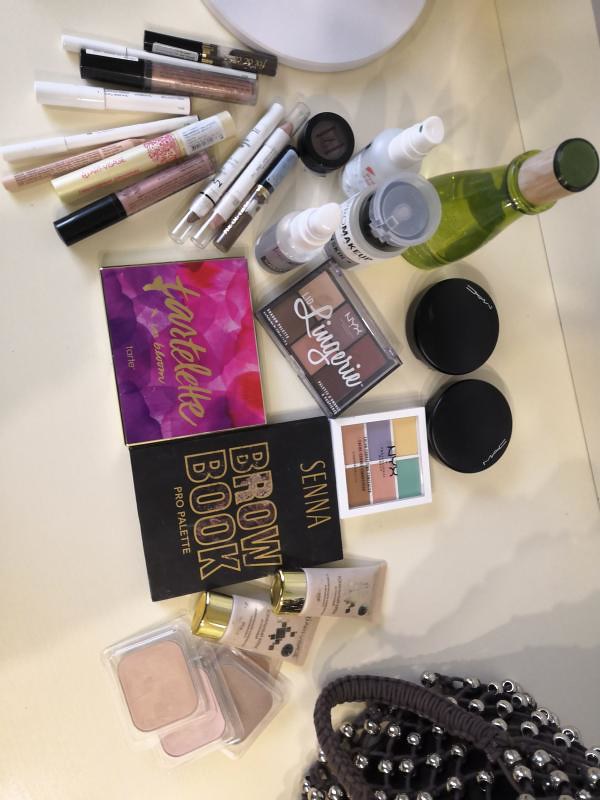This captivating image, taken in portrait mode and spanning a 4x6 frame, showcases what appears to be a vanity area, likely belonging to an individual who enjoys beauty products. The bottom right-hand corner features a stylish woven light handle purse intricately adorned with silver beading, hinting at an elegant touch in the owner's fashion sense. 

The vanity is arrayed with an impressive collection of pristine, untouched makeup items, suggestive of a recent shopping haul. At the top, a selection of lip glosses and what appear to be eyebrow pencils or eyeliners are neatly positioned. There are four distinct sets of palettes: 

1. One vibrant palette in shades of pink and purple, though the brand name is not discernible.
2. A "Brow Book Pro Palette" by Sena, distinguished by its black case with gold lettering.
3. An NYX eyeshadow palette featuring brown and neutral tones.
4. Another compact palette that includes cheerful colors like pink, yellow, and green, likely for eyeshadow and blush.

Additionally, there are two MAC compacts, easily recognizable by their sleek design, and several tubes of concealer, all impeccably arranged. This ensemble of makeup products paints a vivid picture of the owner's diverse and upscale tastes in beauty essentials.